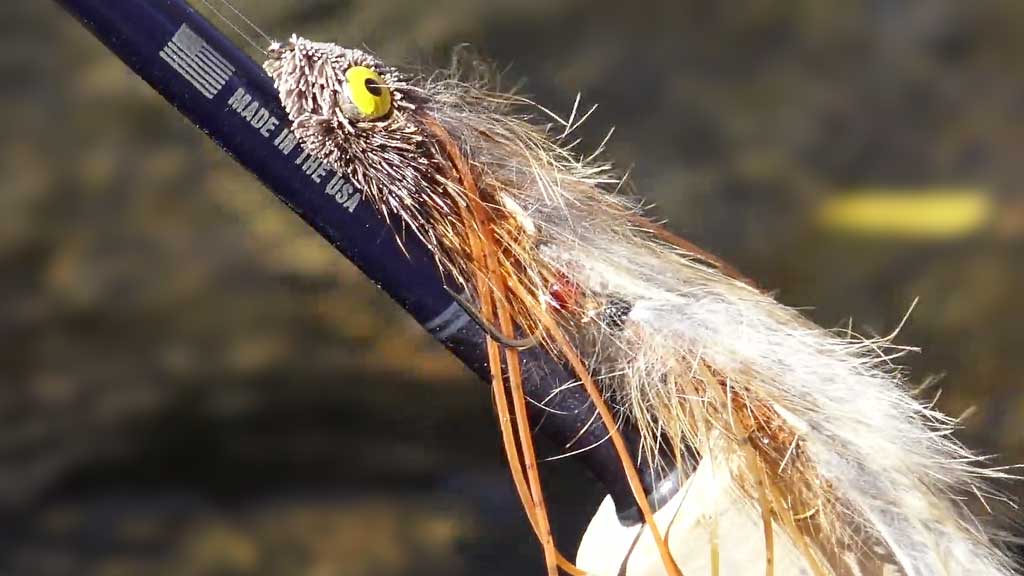The image features a detailed artificial fishing bait. The bait is adorned with a round yellow eye, highlighted by a black pupil, and surrounded by shorter hair-like structures. Emanating from the bait are long, thick orange strings, as well as thin, white, fluffy strands that add to its intricate appearance. About a third of the way down, a silver hook is visible, protruding from the bait. The entire setup rests against a black fishing pole. The fishing pole is marked with a black-and-white American flag and the phrase "Made in the USA" written in white, enhancing the patriotic theme of the image.